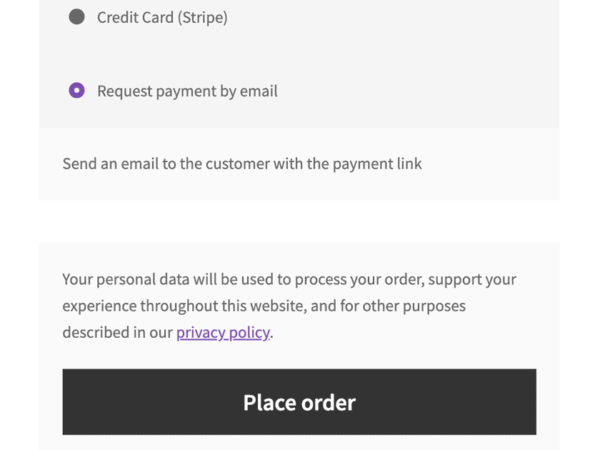The image presented features a structured layout designed for an online payment and order processing interface. Here is a detailed caption:

---

The image showcases a user interface for an online payment system, predominantly featuring shades of gray, black, white, and hints of purple. At the top left of the interface, a light gray background is adorned with a circular black dot next to black font text that reads "Credit Card" followed by the word "Stripe" in brackets. Directly below this section, there is a purple circle with a white dot in its center, accompanied by black font text that says "Raise a request payment by email." This is followed by a lighter gray text that instructs, "Send an email to the customer with the payment link." 

The following segment features a white box, which contrasts sharply with the preceding and subsequent gray sections. Below this white box, returning to the lighter gray background, black font text informs users, "Your personal data will be used to process your order, support your experience throughout this website, and for other purposes described in your own privacy policy." The term "Privacy Policy" is distinctly highlighted in purple font with a purple outline, ending with a period.

At the bottom of the page, a black box is prominently placed, containing the text "Place Order" in white font centered within it. The entire layout is bordered by lighter gray, providing a clean finish to the structured design.

---

This caption provides a detailed and coherent description of the image, emphasizing the visual elements and textual instructions featured.